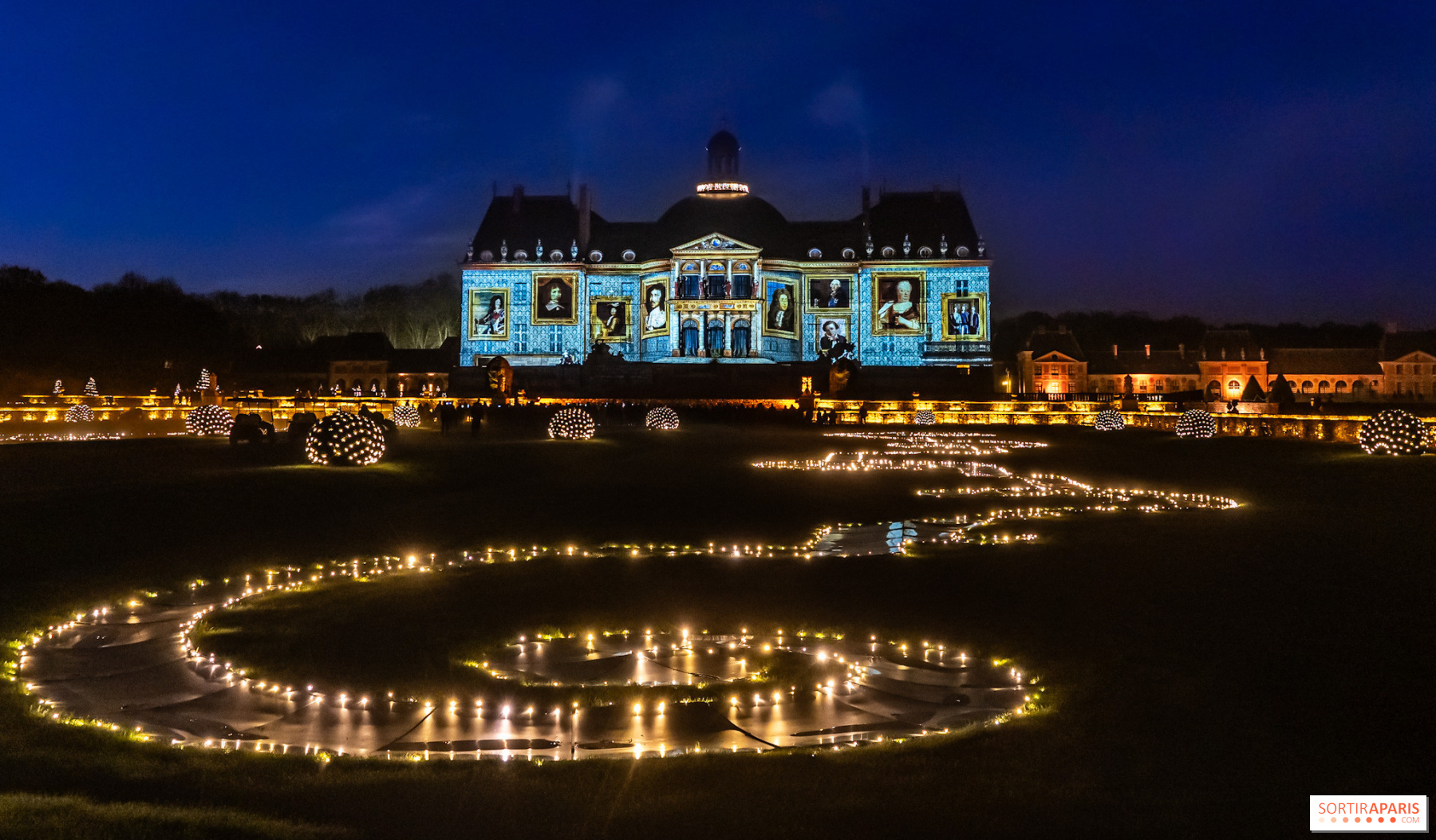This nighttime image captures a highly illuminated house adorned with a myriad of vibrant lights, creating an elaborate light display across the lawn and the house itself. The front yard is decorated with lights that encompass shrubs, making them appear like glowing orbs, and forming intricate swirling patterns that lead towards the house. The house, which exudes an appearance reminiscent of a state or historical building, possibly resembling a castle or a capital, is strikingly covered in light blue projections. These projections showcase large-scale portraits and artistic images, creating a facade that blends photography and artwork, adding an ethereal quality to the scene.

Atop the house and spanning its entire width, the decorations, which also encircle the top structure, enhance the architectural outline with radiant illumination. This seemingly false architectural structure, potentially making the house appear larger and more grandiose, stands out dramatically against the night sky. In the background, dark blue skies frame additional buildings and trees that remain undecorated, providing a contrast to the vivid light display in the foreground. The mix of yellows, blues, browns, and oranges coloring the scene suggests the possibility of an artistic projection or a greatly colorized photo, further adding to the surreal and almost dreamlike visual experience. The presence of subtle signage suggesting Paris hints at the location being a possible tourist attraction, where the building and light display are a focal point for visitors.